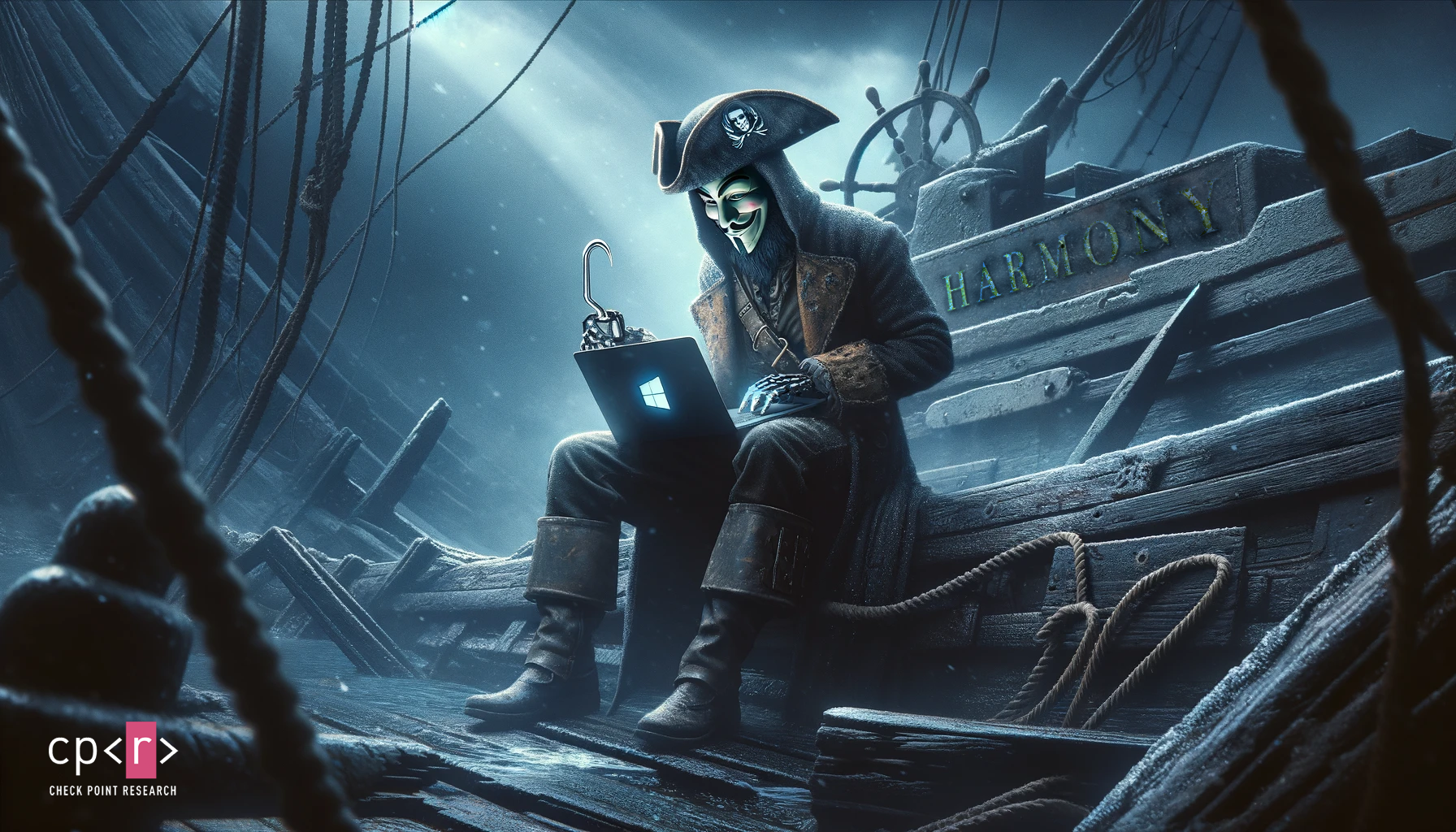In this visually striking, computer-generated image presented by Checkpoint Research, we see a pirate captain sitting on the edge of a dilapidated pirate ship, under the moonlit sky. The captain is adorned in traditional pirate attire, complete with a pirate hat, boots, and a hook for a right hand. Adding a modern twist, his face is concealed by a Guy Fawkes mask, synonymous with the Anonymous movement often associated with 4chan forums. A black laptop, illuminated by a glowing Windows logo, rests on his lap as he uses his left hand to navigate. 

The scene is cluttered with typical pirate paraphernalia—wooden planks, ropes, and an old ship's wheel—reflecting a sense of abandonment. Faded yellow letters spelling "Harmony" appear to the left of his shoulder, hinting at a deeper, perhaps ironic meaning. The subdued palette of dark blues and grays accentuates the sinister, mysterious atmosphere. A caption in the bottom left reads "CP<R>" with "Checkpoint Research" delineated in white and pink text, further anchoring the image's connection to contemporary themes of cybersecurity and hacktivism.